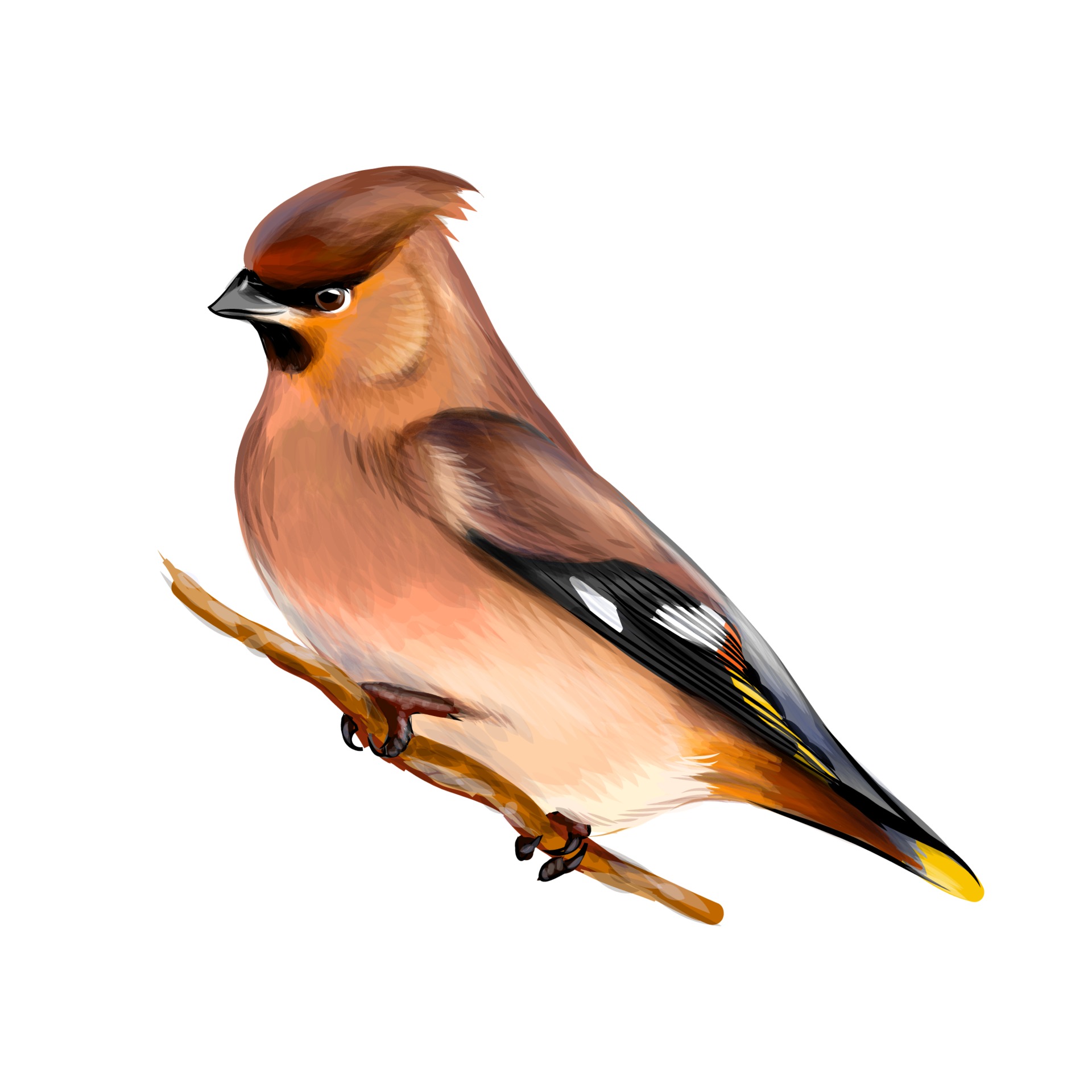The image is a detailed, realistic drawing of a bird perched on a small, slender branch, which appears to almost float against a stark white background. The bird's clawed feet grip the branch tightly, showcasing its black claws. Its legs are pink, contrasting with its black-tipped feathers. The bird's body exhibits a gradient of colors, predominantly reddish-brown with a hint of orange and yellow towards the tail feathers. The wings transition from reddish-brown to black, white, orange, and yellow. The head of the bird, reminiscent of a robin's, is dark brown with some black accents around its eyes and chin, and areas tinged with yellow. The beak is short and black, and the eyes are brown. The depiction is highly detailed and life-like, highlighting the intricate feather patterns and vibrant coloration, set against a bright and clear background that emphasizes the bird's features.